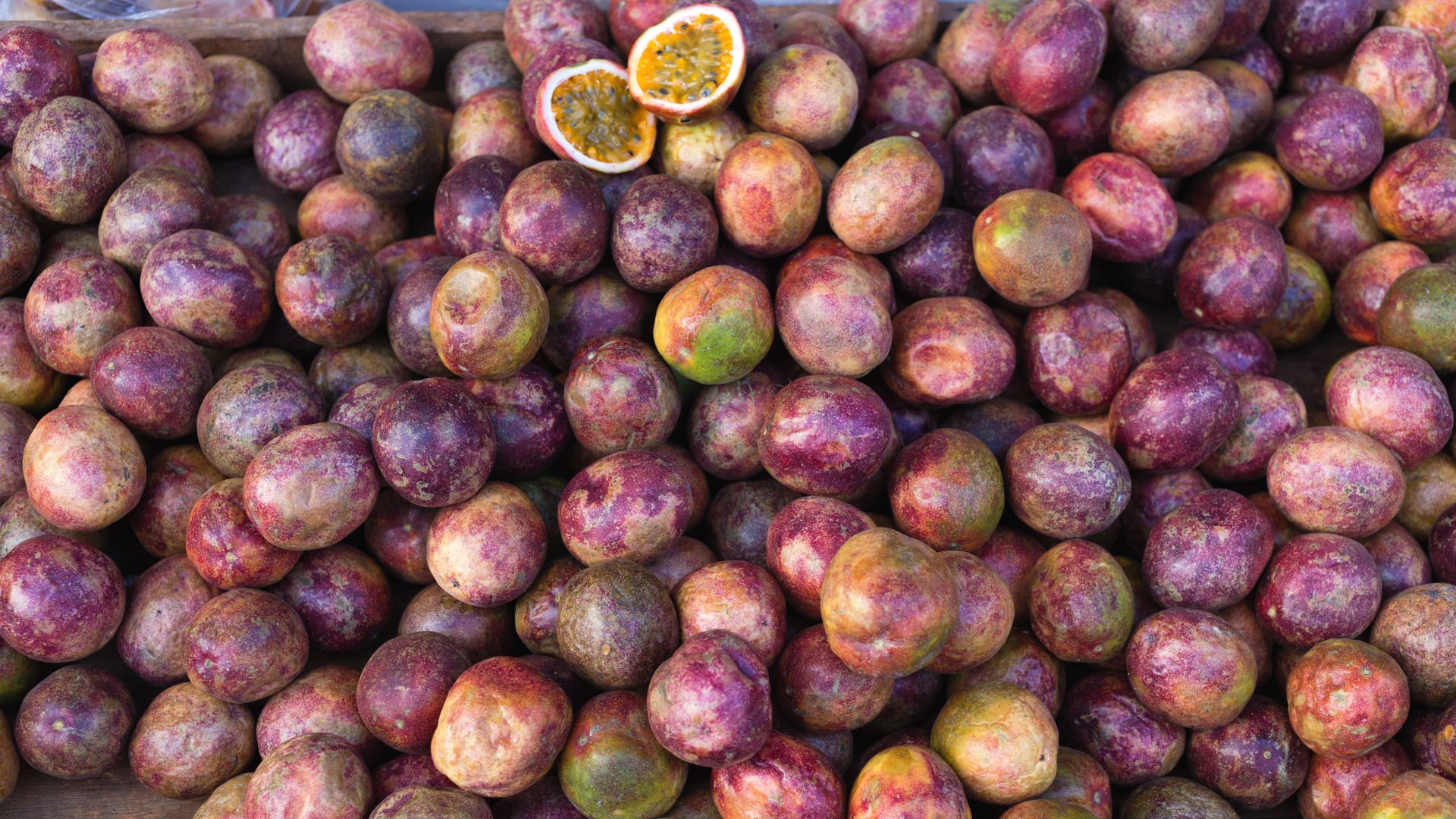This overhead image captures a wooden box brimming with variously colored passion fruits. The fruits are primarily spherical, displaying a rich tapestry of purple splotched with green, yellow, red, and brown hues. Amidst this vibrant assortment, one passion fruit stands out, halved to reveal its interior. The cut fruit shows a thick white rim encircling its yellow, fleshy center, dotted with tiny black seeds. Its central placement in the photograph draws the gaze, contrasting with the mosaic of the other uncut fruits surrounding it.